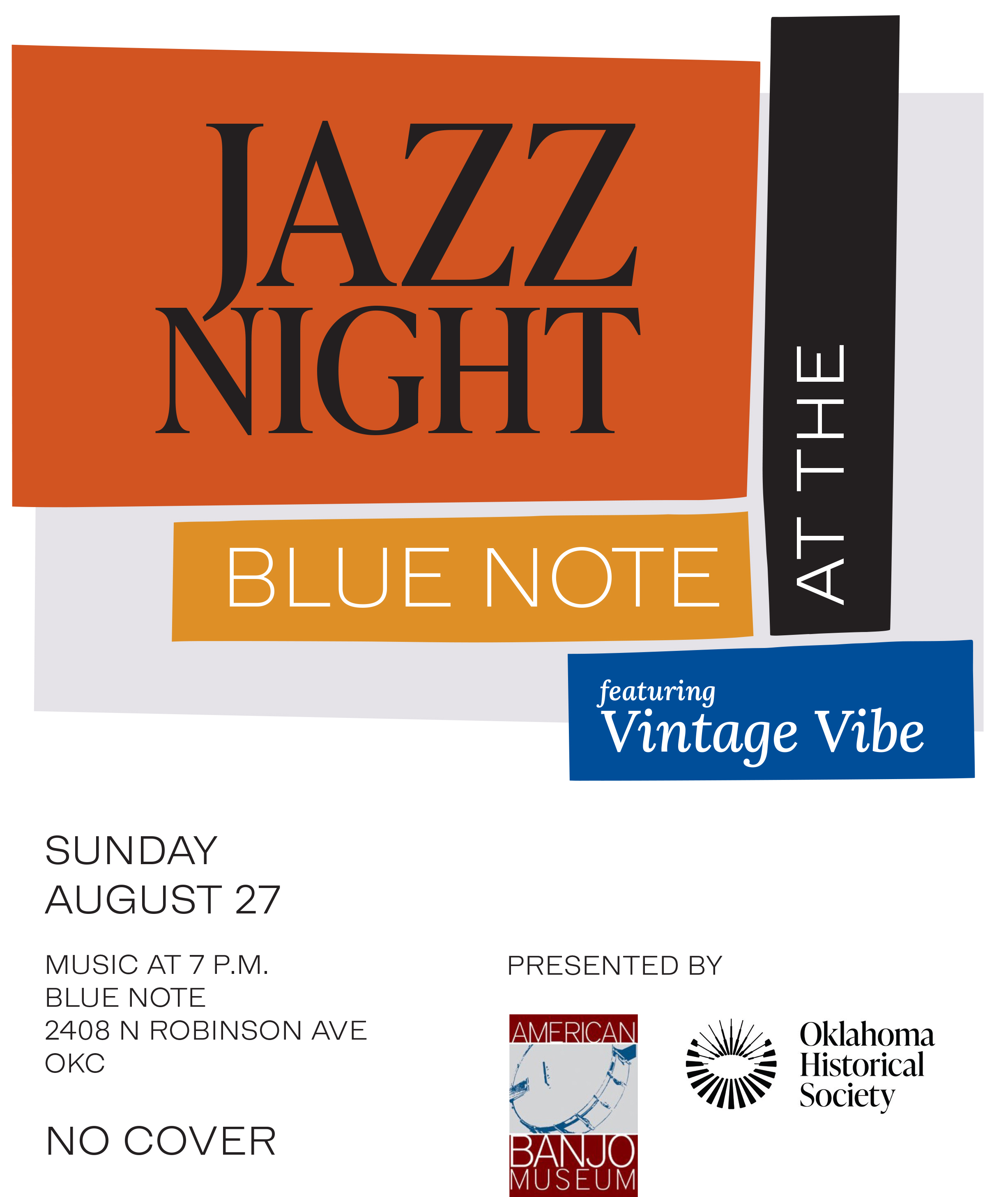The poster for Jazz Night at the Blue Note prominently features vibrant, multicolored text in orange, yellow, blue, and black, announcing "Jazz Night at the Blue Note." Below this main title, the event details are listed in plain text on a white background: "Sunday, August 27th, music at 7pm, Blue Note, 2408 North Robinson Avenue, OKC, no cover." The bottom section of the poster includes sponsorship information, presented by the American Banjo Museum, with their blue and red logo featuring a banjo, and the Oklahoma Historical Society, with a circular logo emblazoned with stripes. The eye-catching design appears to be digitally crafted, likely using design software, with the title prominently positioned in various colored rectangles and "featuring Vintage Vibe" displayed in a blue box in cursive text.